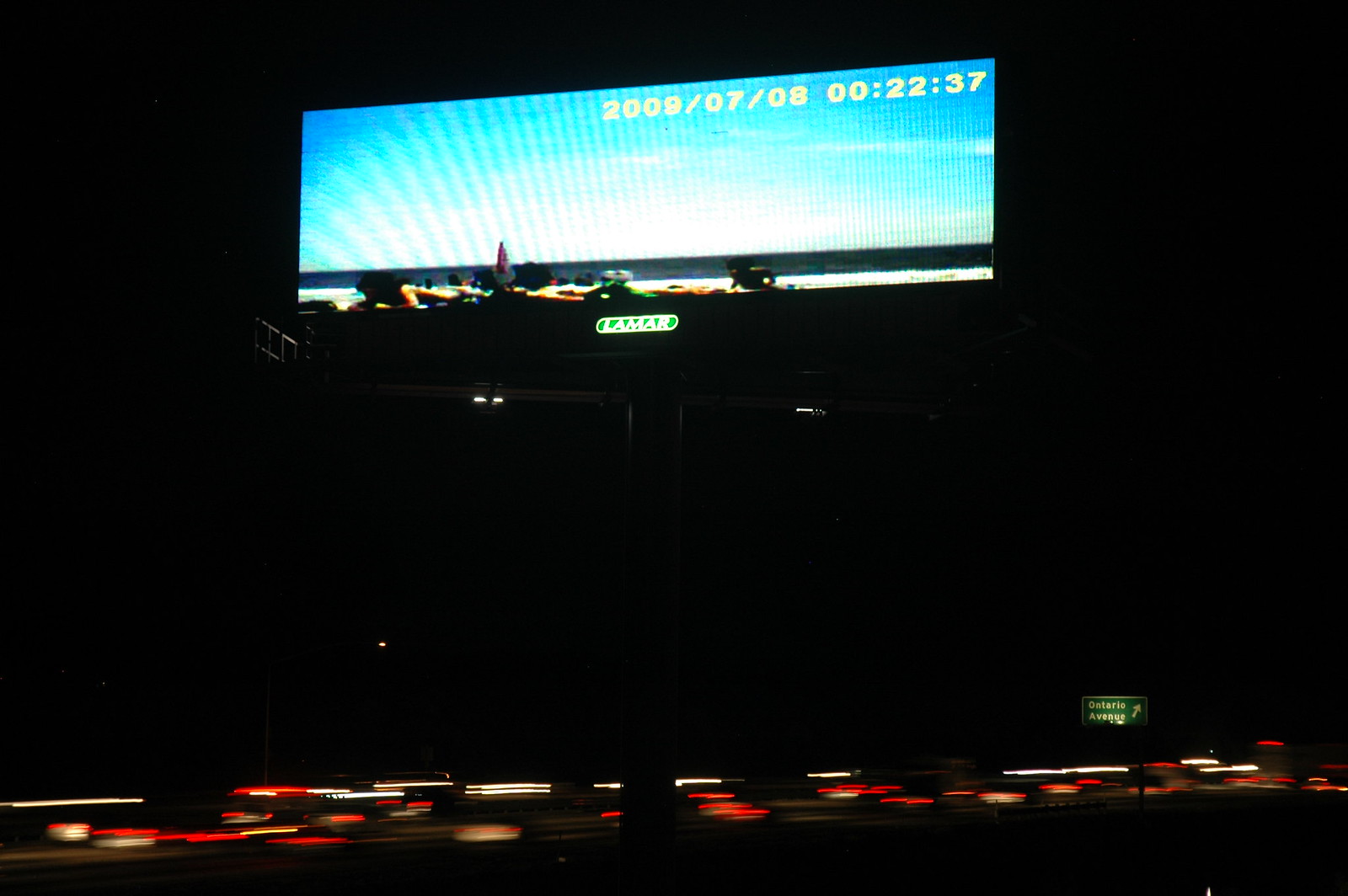The image depicts a rectangular billboard photograph taken at night. The billboard dominates the center of the frame, with the long side extending from left to right. The backdrop is enveloped in pitch-black darkness, highlighting the vibrant illumination of the billboard. The top edge of the billboard features a bluish-aquamarine colored trim. Displayed prominently on the billboard in yellow text is the sequence "2009/0708" followed by "00:22:37."

At the bottom of the billboard, the word "Lamar" is clearly visible, printed in white letters against a green background. Beneath the billboard, a pole slightly visible supports the structure. The lower part of the image hints at traffic activity, with red taillights visible, suggesting vehicles are moving away from the photographer. The overall scene captures the stark contrast between the brightly lit billboard and the surrounding darkness, with subtle hints of nocturnal city life.